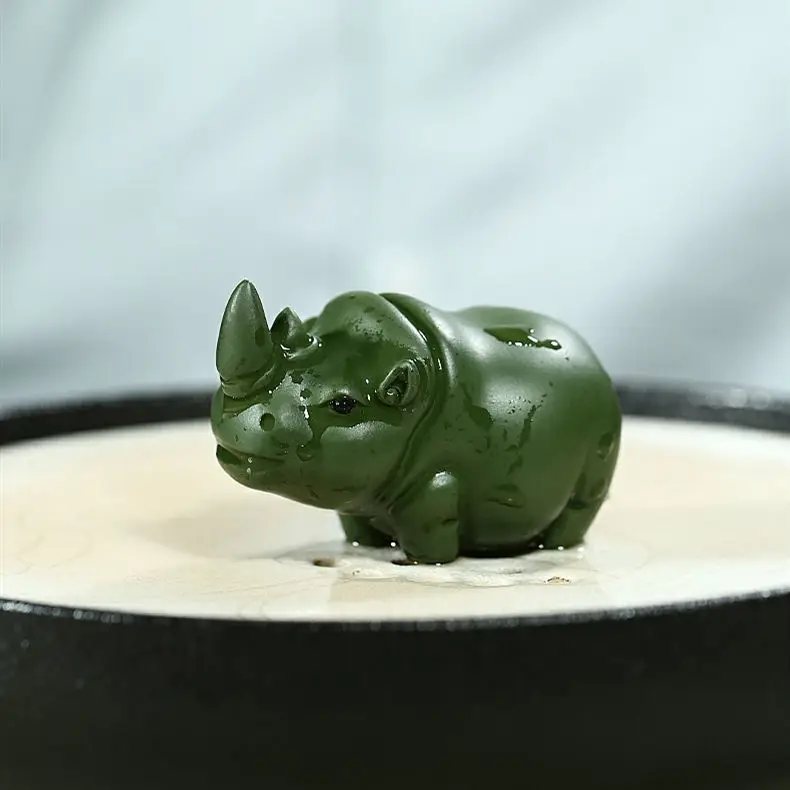A detailed description of the image captures a small, green rhinoceros figurine, likely made of plastic and exhibiting a cartoony design. The figurine is short and stubby, with well-defined small ears, tiny nostrils, a partially open mouth, and black bead-like eyes. The horn is situated at the top of its head. Water droplets are visibly clinging to its surface, with some appearing to run down its side, giving the impression that the rhinoceros is crying. The figurine is submerged in a dense, cream-colored liquid resembling pudding or a thin soup, contained within a black bowl. The background features a blurred, grayish sheet, ensuring the rhinoceros remains the primary focus of the image.